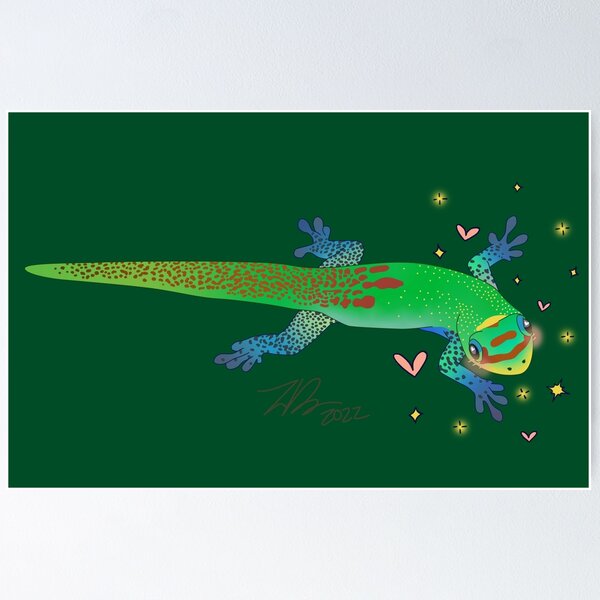This is a detailed illustration of a gecko-like lizard set against a deep dark green background. The lizard, positioned horizontally, showcases a bright green body with a gradient shading, highlighted by distinctive brown spotting that extends along its tail and up its back. The shoulders feature smaller yellow spots, transitioning to prominent reddish-orange markings that run down to the tail. The lizard's legs are primarily blue, fading into white and green, adorned with darker blue spots and each foot displaying four digits with bulbous tips. Its face is distinguished by two red stripes across the forehead, yellow at the nose tip blending into green, and large, expressive eyes that are black, white, and blue. Surrounding the lizard's head and front legs are pink hearts and golden star-like sparkles, adding a whimsical touch to the scene. The illustration is signed "HB 2022" and blends artistic creativity with detailed anatomical representation, particularly in the limbs and facial features.